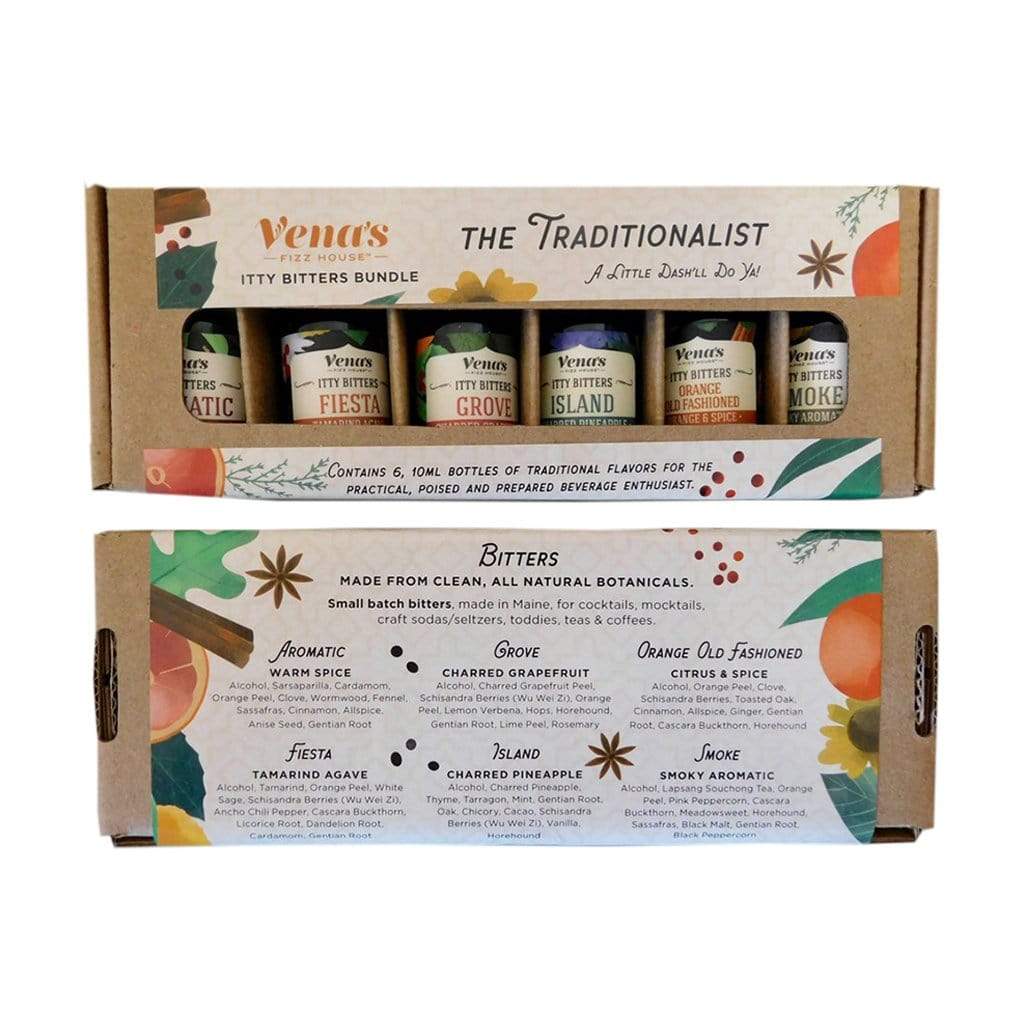The image showcases a product photo of Viva's Itty Bitters Bundle, a collection of six small bottles of bitters, packaged in a cardboard box. This packaging boasts a sticker label adorned with watercolor illustrations of star anise, herbs, cinnamon sticks, citrus, and flowers, evoking a botanical and herbal aesthetic. The front of the box features a cutout revealing the six 10ml bottles inside, labeled for the "traditionalist, a little dash will do ya." The label further details that the box contains six traditional flavors intended for the practical, poised, and prepared beverage enthusiast. 

On the back of the package, the bitters are described as being made from clean, all-natural botanicals in small batches in Maine, suitable for cocktails, mocktails, craft sodas, seltzers, toddies, teas, and coffees. Each variety is briefly described along with its key ingredients: Aromatic Warm Spice, Grove Charred Grapefruit, Orange Old-Fashioned Citrus and Spice, Fiesta Tamarind Agave, Island Charred Pineapple, and Smoke Smoky Aromatic. While the detailed ingredient lists are hard to read, they hint at a thoughtful blend of unique flavors, adding to the appeal of this meticulously designed and artistically presented product.